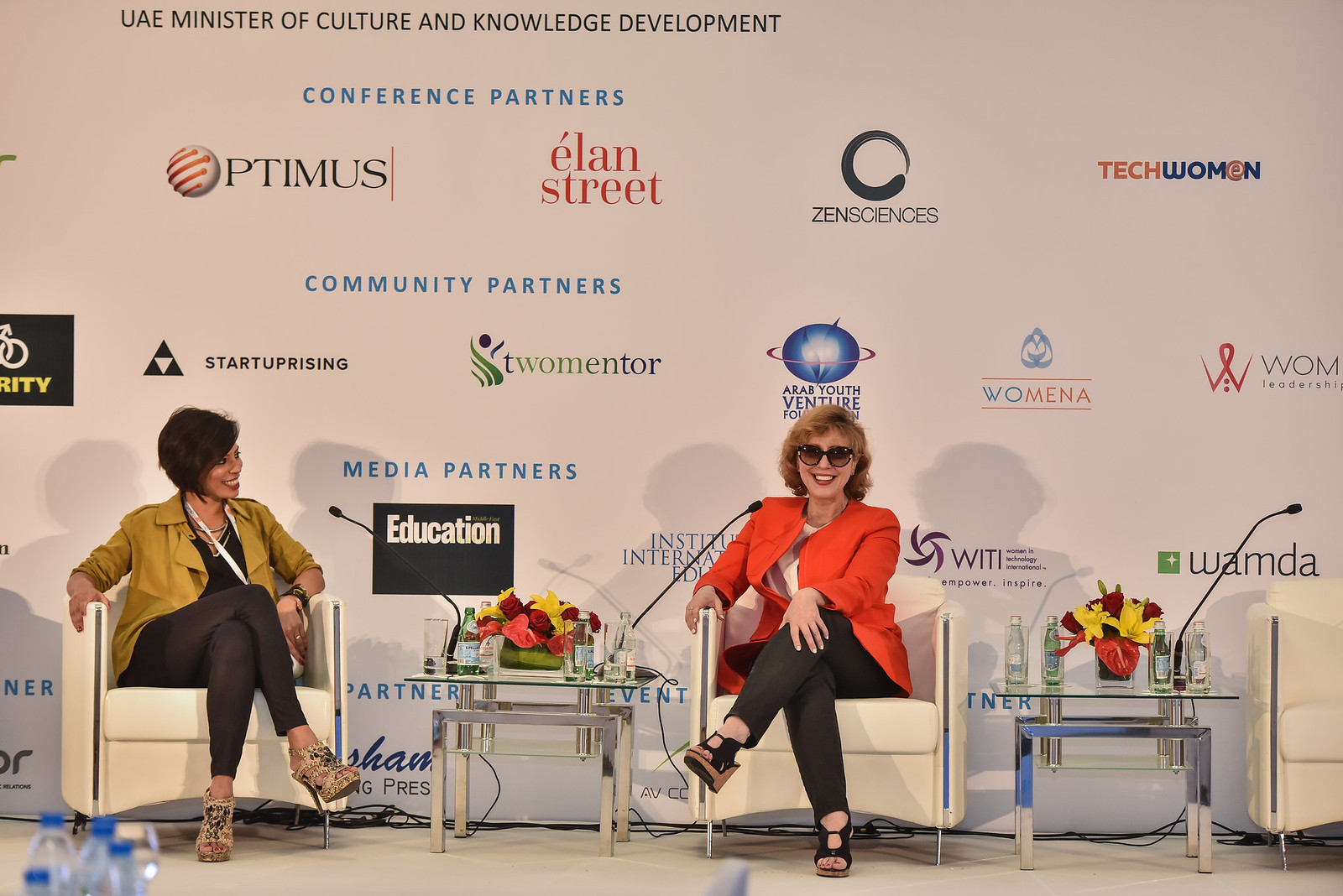The landscape-oriented color photograph depicts an interview stage set with three white chairs. Two women are seated in the chairs—one in the center and one to the left. The woman in the center, who appears to be the moderator, is wearing an orange blazer, black pants, and tinted sunglasses. She is seated with her legs crossed, smiling, and looking directly at the viewer. The woman on the left is clad in a yellow-tan blazer over a black blouse, black leggings, and high heels; she has dark hair and is facing the moderator while smiling. In front of each, silver coffee tables feature black microphones extending toward the women. The stage has a tan floor and a backdrop adorned with multiple sponsor logos, including names like Tech Women, Pitmas, Lane Street, and Optimus. Scattered water bottle tops are visible on the stage floor. The overall style is photographic representationalism, realism, capturing this educational or professional event.